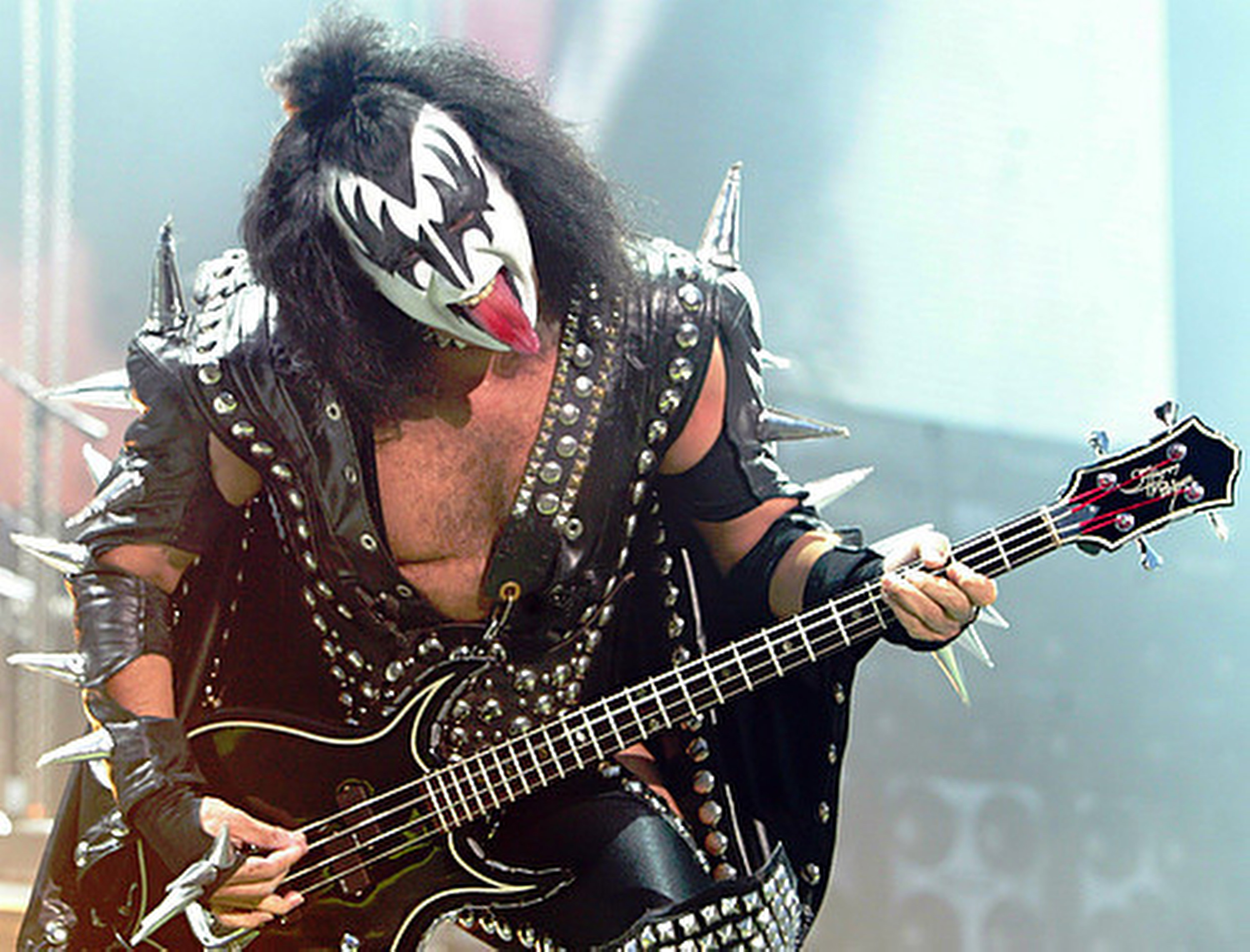The photograph captures Gene Simmons, the iconic rock star from the band KISS, during a live concert performance on stage. Central to the image is Simmons in full KISS garb, characterized by his distinctive white face paint with black bat-wing patterns around his eyes. His expression is intense, with his eyes wide open and his mouth agape, revealing his yellowed top row of teeth, and his tongue defiantly sticking out. He sports shaggy, black hair styled in a half-updo, half-down manner resembling a straw-like texture.

Simmons' elaborate outfit is made of black leather adorned with silver studs, buttons, and spikes that accentuate his theatrical stage presence. His chest is bare, flaunting his muscular arms that are decorated with metallic spikes. His ensemble is completed with black leather pants and a cape. The black electric guitar he wields, which has hints of green and a white outer lining, adds to his formidable rock persona.

The stage background is slightly blurred but noticeable enough to hint at a drum set, sound equipment, and possibly a screen. Despite the professional quality and clarity of the photo, no audience or other band members are visible in the frame. The ambiance and details suggest that this vibrant, high-energy shot was captured during a dynamic segment of the concert, where Simmons is fully immersed in his performance, captivating the unseen crowd with his legendary showmanship.